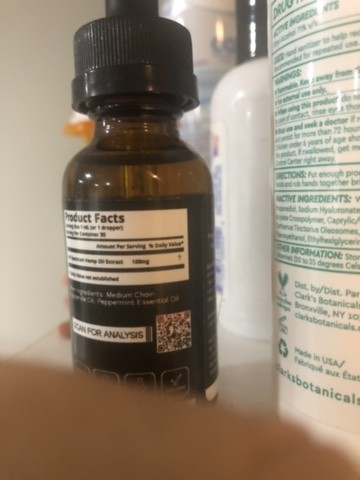This photograph features the back view of a small glass container equipped with an eyedropper. The container, holding approximately one ounce of liquid, is accompanied by a black plastic dropper and a clear tip. The label on the bottle includes a "Product Facts" section, though the print is too fuzzy to decipher the details. Additionally, a small QR code is visible beside some partially obscured text mentioning "analysis." A large thumb partially obstructs the view, contributing to the difficulty in reading the label.